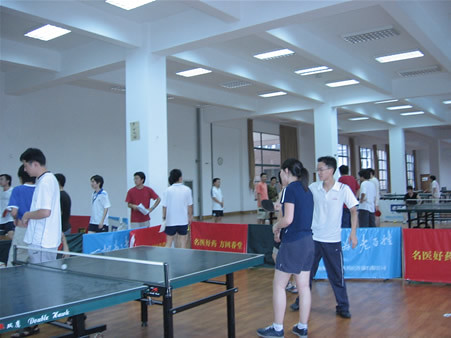The photograph, rectangular in shape and of moderate quality, appears to be taken with an older style camera in a spacious room with a high ceiling illuminated by square fluorescent lights, reminiscent of those in a gymnasium or school. The room features multiple support pillars and is set up for a competitive ping-pong event, evidenced by the numerous ping-pong tables scattered throughout and various colored banners—red and blue—delineating different areas. The gym floor is bustling with activity, as approximately 15 to 20 individuals, predominantly in their 30s or 40s and of Asian descent, move between the tables. Significant details include a woman in a blue Adidas shirt, standing with a blue ping-pong table in front of her, surrounded by people in white shirts preparing for their matches. The bottom left corner showcases a classic green ping-pong table with a white net, highlighted by various signs with Chinese or Asian lettering throughout the room. Despite not seeing anyone actively playing at the moment, the photograph captures the lively anticipation and organization of the event.